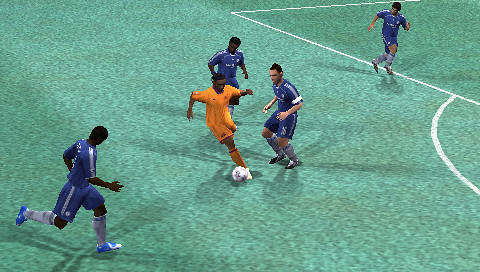In this FIFA soccer game, a vibrant green AstroTurf field sets the stage. At the bottom of the image, a classic white soccer ball is in motion. The central player, skillfully dribbling the ball, stands out in an orange shirt. Surrounding him are four defenders donned in blue shirts, attempting to close in on him. The goal area, marked by distinct white lines, is positioned towards the right side of the field, creating a clear target for the offensive play.